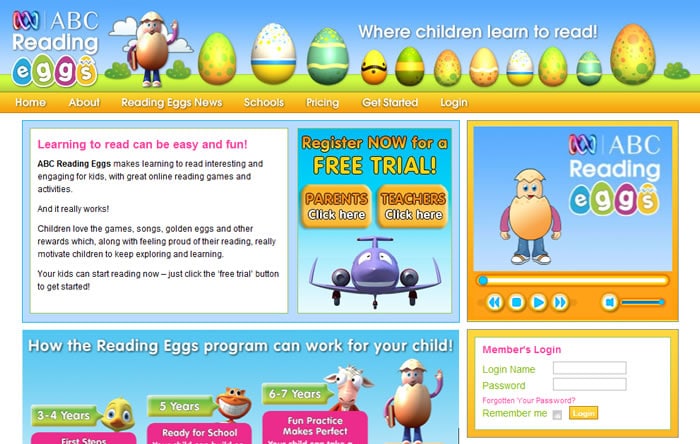This is an image of a cropped screenshot from the website ABC Reading Eggs, an online platform designed to assist children in learning to read. The top header of the website features a cartoon-like illustration of a sky and grassy area, adorned with eggs of varying sizes lined up horizontally. Above these eggs, a large white text reads "Where children learn to read." On the far left, an egg character waves while holding a book, next to the ABC Reading Eggs logo displayed at the top.

Beneath the header, a yellow navigation bar spans the width of the image, featuring links for "Home," "About," "Reading Eggs," "News," "Schools," "Pricing," "Get Started," and "Log In." Below this bar, a large blue section occupies much of the center. On the left of this section, a white box contains bold pink text stating, "Learning to read can be easy and fun," followed by a detailed description of the services offered by the website.

To the right, a large square box with a blue background displays a cheerful purple plane with a smiley face, illustrative of clipart. Above the plane, large yellow text invites users to "Register now for a free trial." Below this message, two buttons are visible: one labeled "Parents click here" and the other "Teachers click here."

On the far right of the blue section, a video player box is labeled "ABC Reading Eggs." The player includes standard control buttons such as stop, rewind, play, and a volume icon. At the bottom right corner, a white box with a yellow border, labeled "Members Login" in pink at the top left, provides input fields for login name and password. Below these fields is a purple hyperlink for "Forgot your password," followed by a "Remember me" checkbox and a small yellow "Login" button to complete the login process.